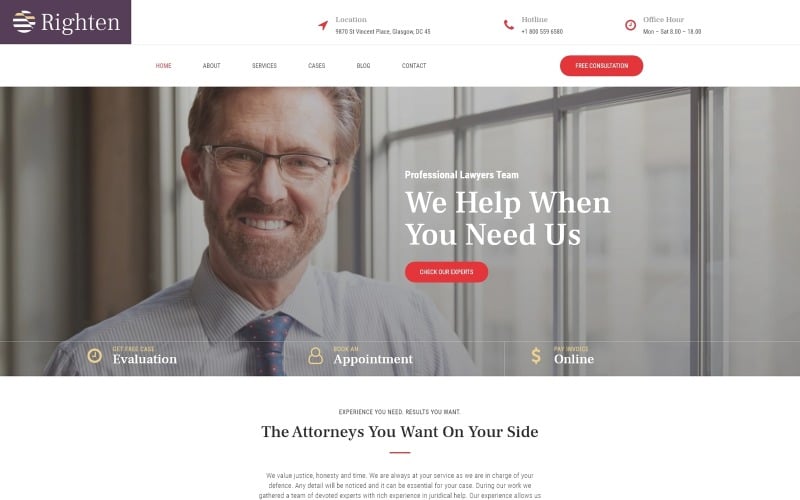This is a screenshot of a website called "Rightin." In the top left corner, there's a darkish purple rectangle featuring the word "Rightin" in white text. To its left, there is a circular symbol with purple stripes. The top right portion of the circle appears cut and shifted upward, giving it an incomplete look. 

The rest of the banner at the top is white and includes three pieces of information: "Location," "Hotline," and "Office Hour." The specific details under "Location" and "Hotline" are small and hard to read. The "Office Hour" segment mentions "Monday to Saturday 8 to something," but the closing time is unclear due to the small font size.

Below the banner, there are six tab options: "Home," "About," "Service," "Cases," "Blog," and "Contact." The "Home" tab is selected and highlighted in red, while the others are in black. To the right of these tabs, there is a red button with white text that reads "Free Consultation."

Beneath these options, there is a picture of a middle-aged man with reddish-brown hair, a beard, and glasses. He is wearing a collared shirt paired with a blue tie that has red polka dots. To the right of his image, the white text says "Professional Lawyers Team. We need us. We help when you need us." Below this text, there is a red button with white text stating "Check Out Our Experts."

At the bottom of the image, it reads "Evaluation," "Appointment," and "Online," indicating three different service options. Finally, there is a blurb that says, "The attorneys you want on your side," followed by a small, hard-to-read paragraph.